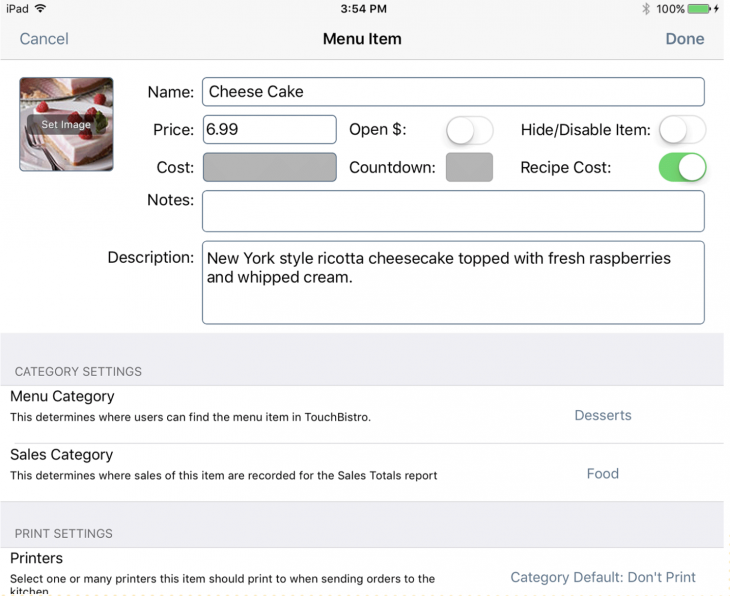A detailed screenshot of an iPad display, showcasing an order being placed via a digital menu. The interface is framed by a light gray border with various status indicators along the top edge, including the black "iPad" label on the upper left, black Wi-Fi signal bars, and the time reading 3:54 PM centered at the top. On the right, the screen shows a gray Bluetooth symbol and a fully charged battery at 100%, highlighted in green with a lightning bolt indicating it's connected to a charger. 

In the bottom left of the screen, there's a light blue "Cancel" button. Centrally aligned, "Menu Item" is written in black with the "Done" button in light blue on the right. The main content below this section displays the item being ordered – a slice of white cheesecake placed on a white plate accompanied by a silver fork. Four red raspberries rest on top of the cheesecake with an additional one placed on the plate.

Adjacent to the image are several interactive fields. The first label is "Name," which has been filled with the word "Cheesecake." Below that, the "Price" field displays "$6.99." To the fields' right are two toggle switches; "Open and a dollar sign" and "Hide-disable item," both unselected with white sliders. Below the price, the "Cost" and "Countdown" fields appear grayed out and inactive. Further down, the "Recipe cost" toggle is activated, showing a green slider. 

The bottom portion includes text boxes labeled "Notes" and "Description." The description reads: "New York style ricotta cheesecake topped with fresh raspberries and whipped cream." The "Category Settings" section outlines two subsections: "Menu Category," listing the item under "Desserts" in light blue, and "Sales Category," categorizing it under "Food."

Additionally, "Print Settings" and "Printer" sections indicate the default category with the instruction "Don't print." The entire background of the interface is clean white, emphasizing clarity and ease of use.